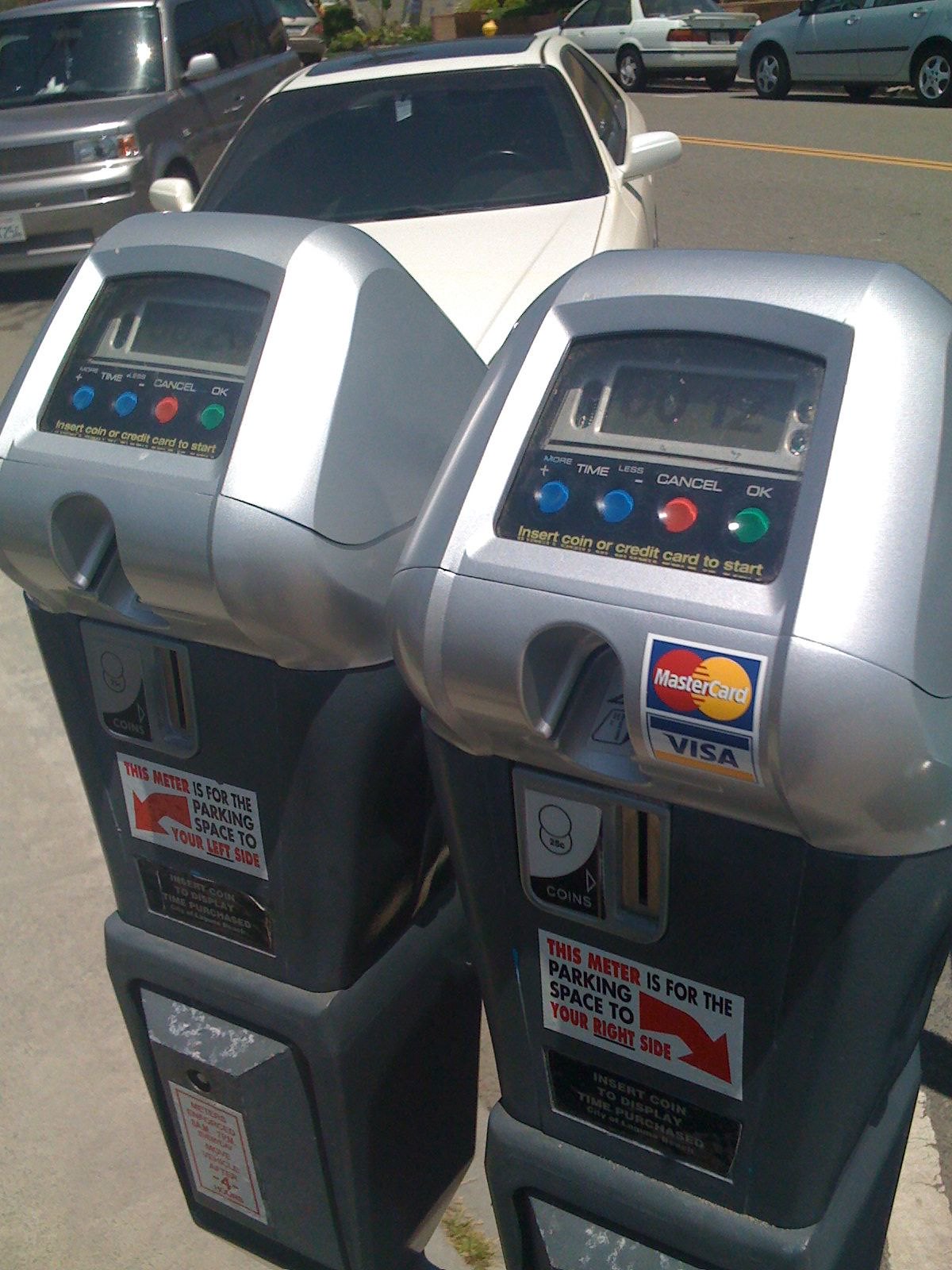The photograph prominently features two digital parking meters mounted side-by-side on a single pole, each displaying LED screens with time readings—12 minutes on the right meter and 26 minutes on the left. Both meters accept MasterCard and Visa for payment and are equipped with credit card slots and coin slots, providing versatile payment options. They feature several interface buttons, including plus and minus buttons for adjusting the time, a red cancel button, and a green OK button. The meters have instructional red arrows pointing to the corresponding parking spaces, with the right one indicating "this meter is for the parking space to your right side" and the left one for the "left side," mounted on a white bracket.

In the background, you can see a gray SUV and a white car facing toward the camera, parked on the same side of the road as the meters. Across the road, a white car and a bluish-aqua car are positioned facing away from the camera. Additionally, a distant building and surrounding shrubs can be seen, suggesting a roadside setting. The sturdy metal frames of the meters contrast with their more plastic-like tops, adding to the modern digital design aesthetic.